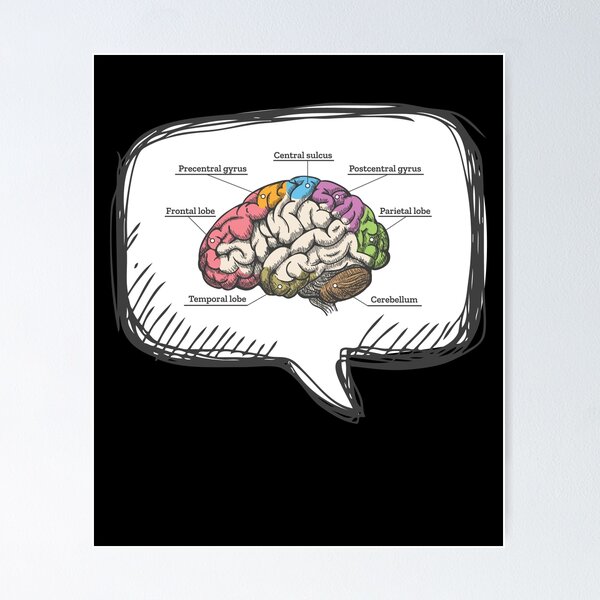The image portrays a human brain diagram inside a white speech bubble with a black, sketch-like border, set against a black background. Various regions of the brain are color-coded and labeled with lines pointing to them. On the lower left, the pink-highlighted area is labeled "Frontal Lobe." Moving upwards on the left side, an orange section is marked as "Precentral Gyrus." The middle top blue segment denotes the "Central Sulcus." The upper right side features a purple area labeled "Postcentral Gyrus." The "Parietal Lobe" is highlighted in green on the lower right, while the "Cerebellum" is depicted in brown at the bottom right. Additionally, the "Temporal Lobe" is indicated in army green from the middle to the lower left side. The image uses a variety of colors—pink, orange, blue, purple, green, and brown—to distinctly highlight and label each brain region within the speech bubble.